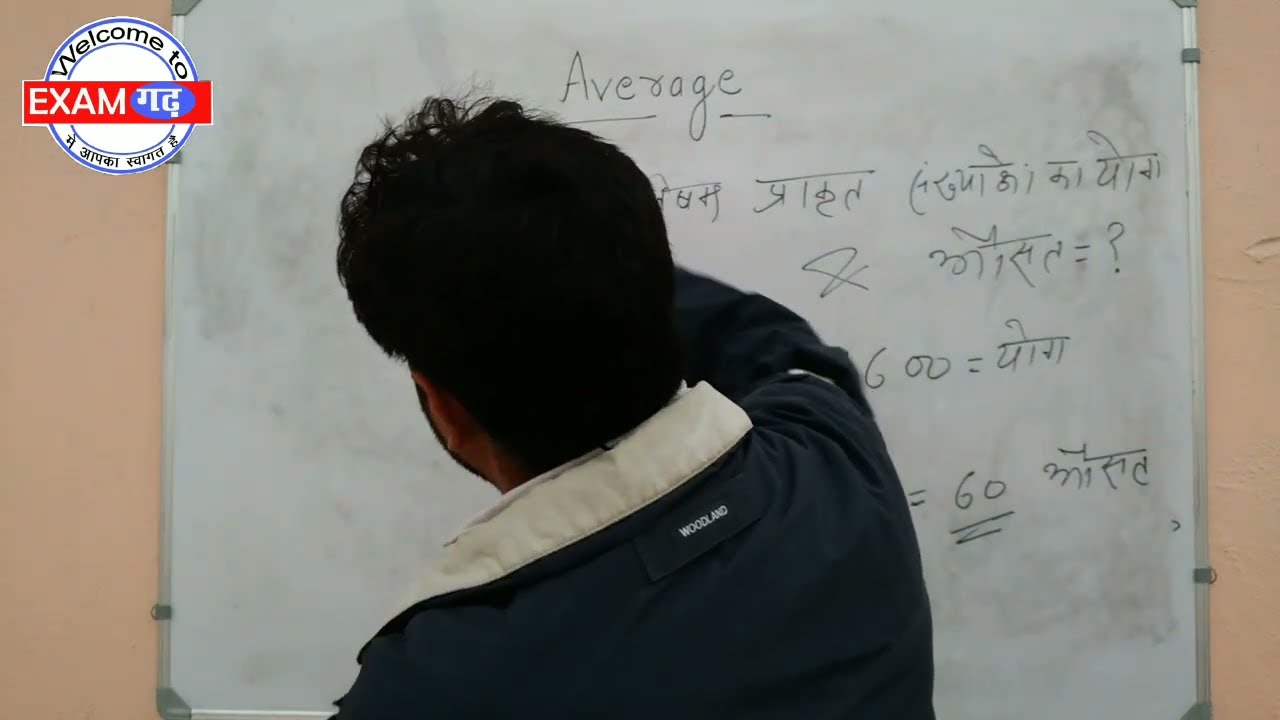The image captures the back view of a young man, possibly a student or teacher, engaged in writing on a small whiteboard, approximately 5 feet by 4 feet, in a classroom setting. He is wearing a dark-colored jacket with a light cream or tan collar, featuring a tag on the back that reads "Woodland." His short, dark hair is visible as he writes with his right hand. The whiteboard is positioned against a beige-colored wall, framed in silver, and covered in various black markings, including mathematical formulas and text. Prominently, the word "AVERAGE" is written at the top of the board. In the top left corner of the image, an overlay features a circular logo with a blue outline, a white background, and a red band across the middle that says "EXAM" in white letters, with "WELCOME TO" above it. The image has an academic atmosphere, filled with intricate details and text that includes foreign languages.